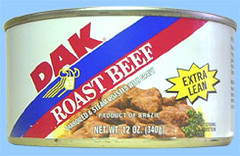The image depicts a predominantly white can of food approximately 3 inches high and 6 inches wide, featuring a distinct silver ring at the top. The can's label showcases a bold red text "GAK" at the top left, followed by a blue stripe below it. Within a prominent red stripe, the label highlights the text "Roast Beef" in bold white letters. An image of the food, comprising brown roast beef accompanied by a green herb garnish, is prominently displayed beneath the text. To the left, in an attention-grabbing impact background, the label emphasizes "Extra Lean" within a yellow circle. The can also includes weight information at the bottom, specifically "Net Weight 12 oz (340 grams)" in white text. The entire label is bordered by gold accents at the top and bottom.